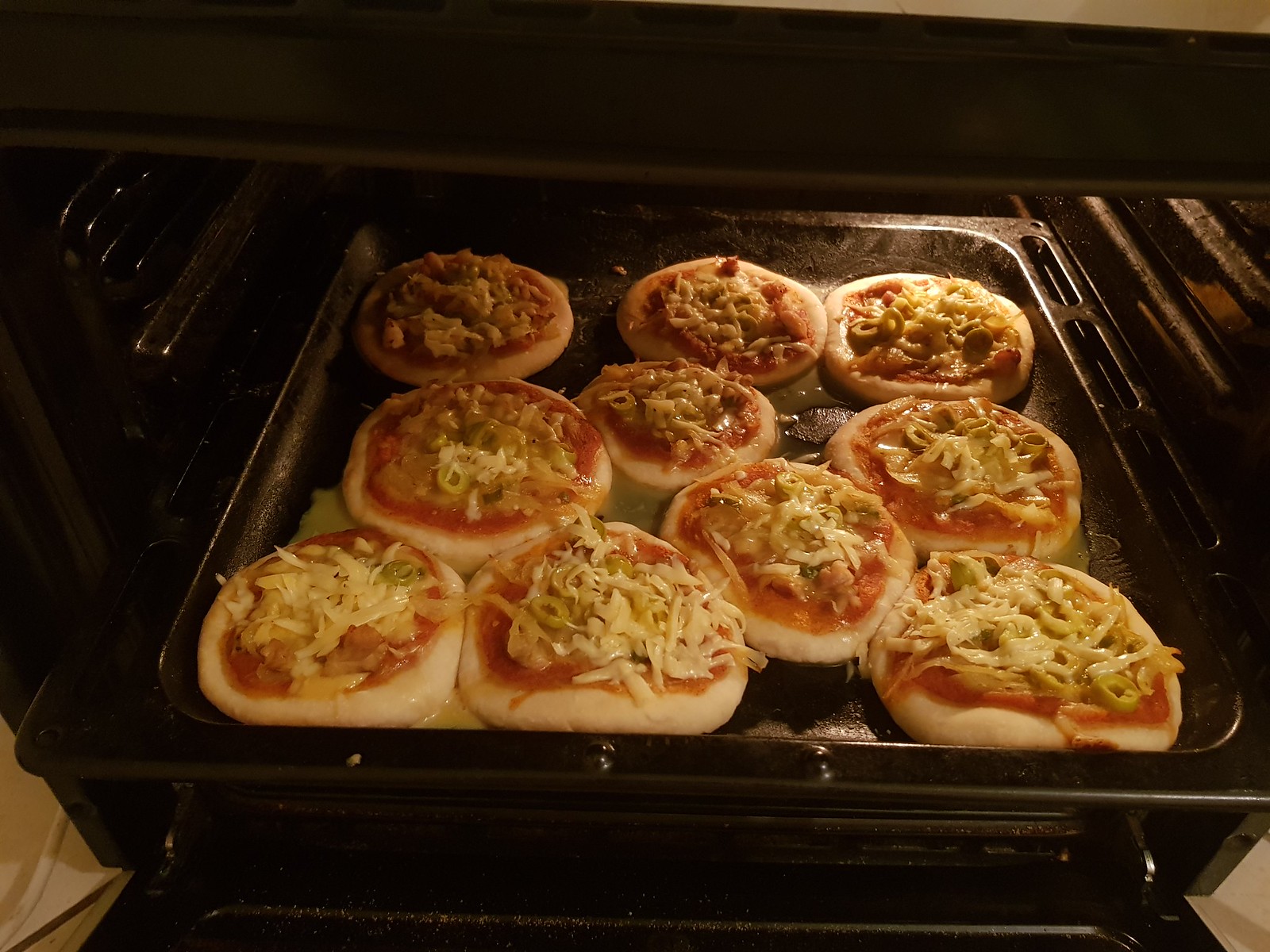This horizontally oriented image, taken from a top-down perspective within a kitchen, showcases the interior of an oven with its door partially open. The oven's interior, primarily black in color, is dimly lit, with only one functioning light on the right side illuminating the scene. Inside the oven sits a slightly deep, black pan containing ten small, circular dough items resembling personal pan pizzas. Each pizza features a layer of red sauce, topped with stringy grated cheese, and garnished with slices of green jalapeno peppers. Notably, some of the dough pieces have a brownish-white coating, possibly flour, and appear to have fluid seeped underneath them, creating a yellowish residue at the bottom left corner of the pan. The overall setup appears somewhat haphazard, highlighting the casual, unrefined placement of the pastries within the pan.